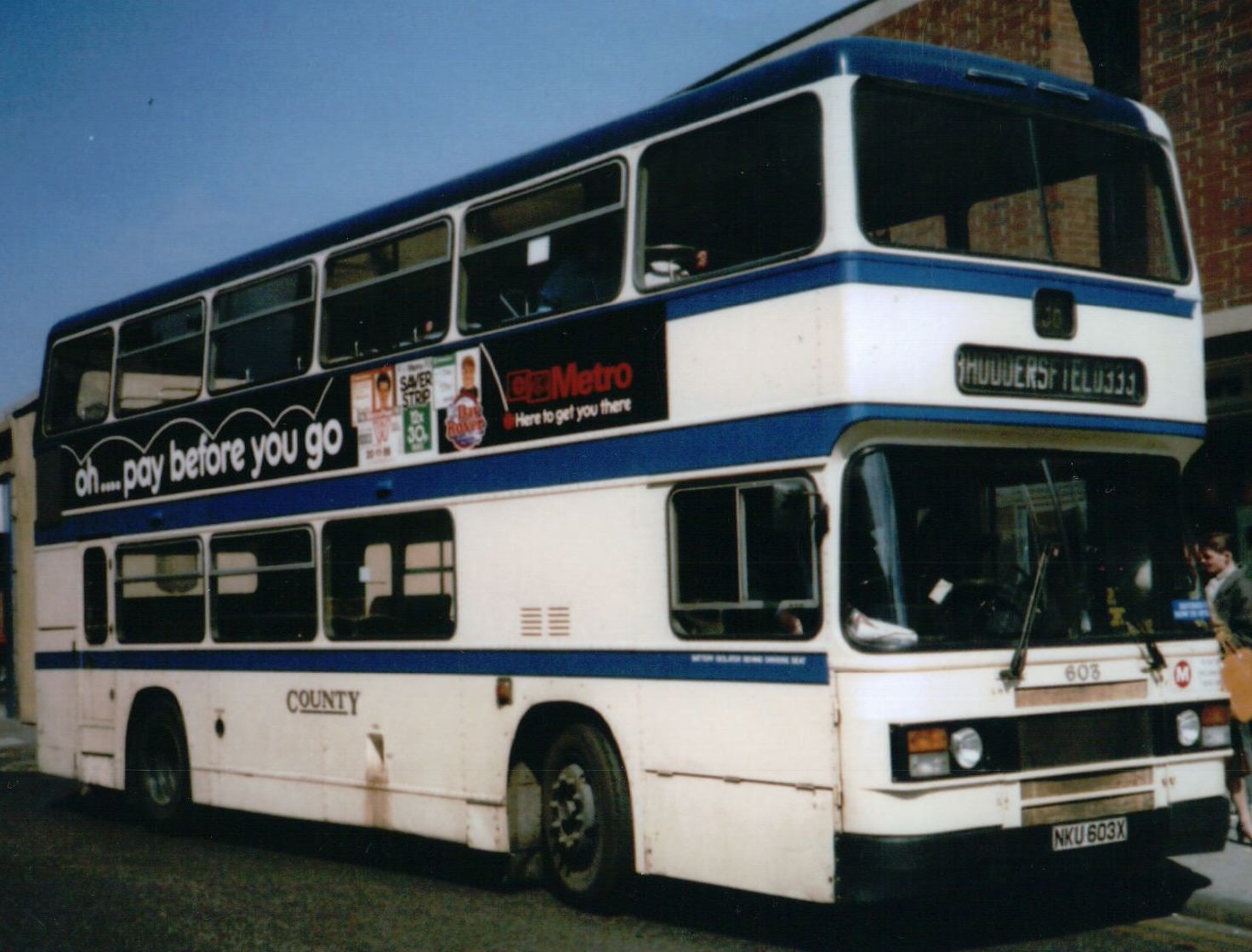The image features a predominantly white double-decker bus with dark blue stripes—and a blue roof—parked on a road under a very blue sky. The bus is adorned with various advertisements; on the blue section near the lower level, the text reads "Pay Before You Go," accompanied by the slogan "Metro, here to get you there." A detail on the side of the first story mentions "county" underneath the windows. At the front, the license plate, inscribed with "NKUS 603X," is set against a white background with dark letters. Passengers are seen lined up to board the bus, and a silhouette of the driver is visible behind the wheel, seated on the right-hand side, indicating that this scene likely takes place in a country where vehicles drive on the left. In the background, one person can be seen standing on the sidewalk to the right of the image.